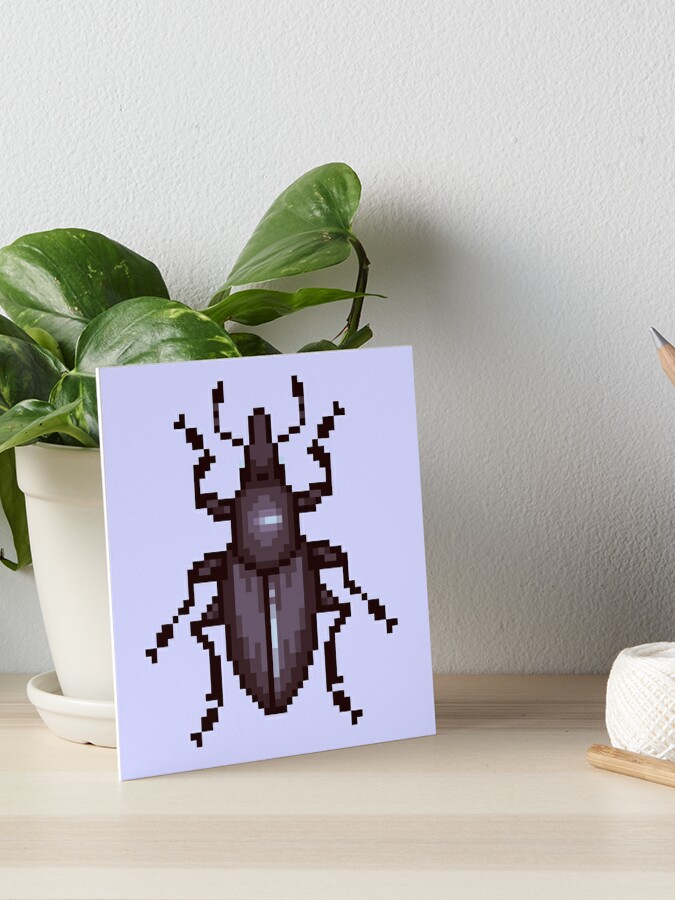The photograph captures a finely detailed image featuring a pixelated representation of a beetle. The artwork, resembling a black or dark grey beetle with a computer game-inspired pixelated design, rests atop a very light, almost white, wooden surface. This card leans against a white or off-white, cream-colored pot that houses a green plant with sword-shaped leaves. The plant's planter includes a matching saucer underneath, contributing to the minimalistic yet inviting aesthetic. Positioned to the right of the image, albeit partially cut off, is a cream-colored object that could be cream-colored yarn or a pencil. The photograph emphasizes the pixelated beetle artwork, creating a striking contrast against its simple, white background, while the surrounding elements enhance the overall composition without detracting from the central visual focus.